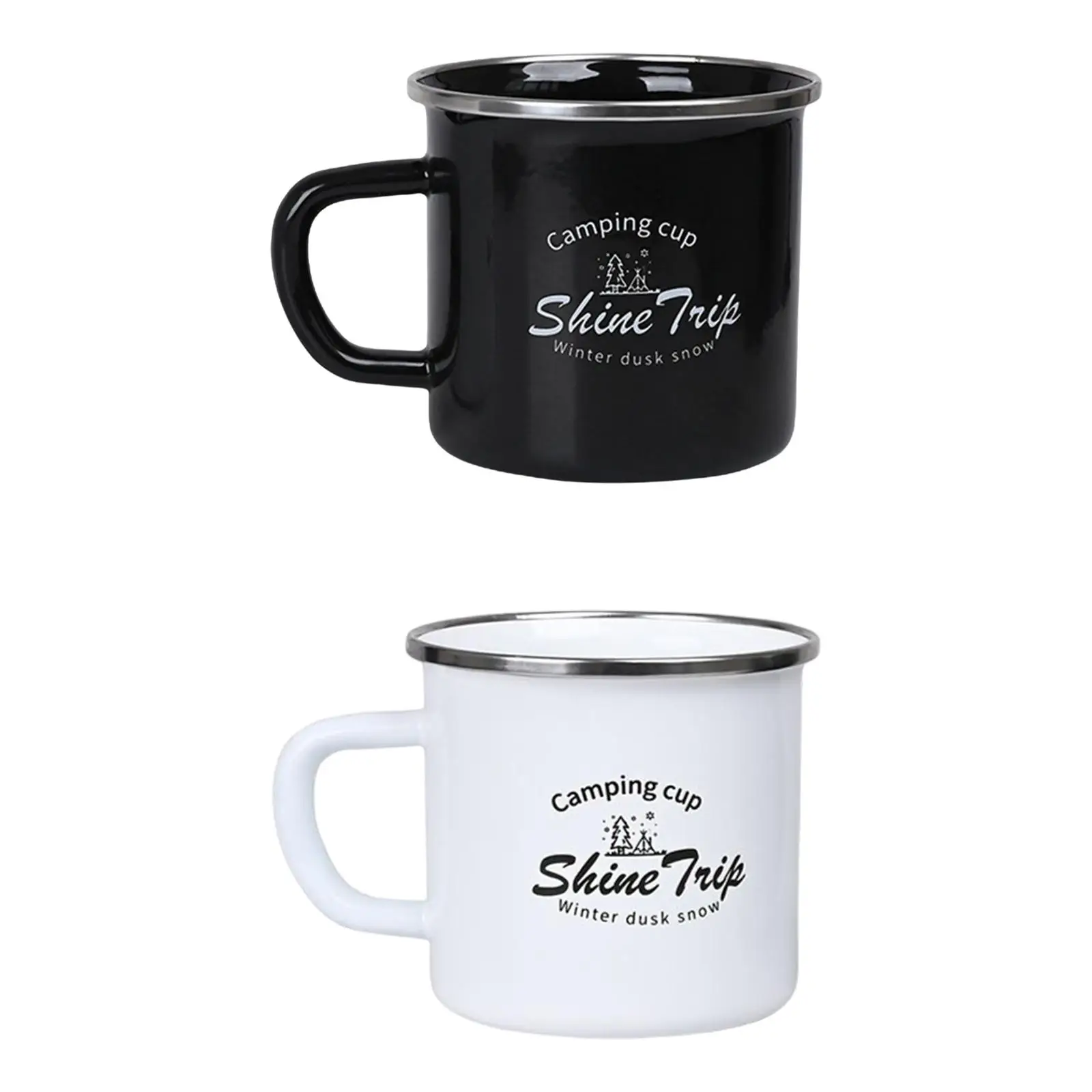The image features two identical coffee mugs, each with a reflective silver rim and a glossy finish. The top mug is black with white text, while the bottom mug is white with black text. Both mugs have the same design elements: at the center, they boldly state "camping cup" in uppercase letters. Beneath this, a small, simple graphic depicts a tent and an evergreen tree. Further down, in cursive, they read "shine trip," followed by the phrase "winter dusk snow" in smaller lettering. The mugs' reflective silver rims gleam, especially on the black mug, which seems to catch and reflect more light. The image has a white or neutral background, highlighting the mugs' detailed designs and reflective properties.